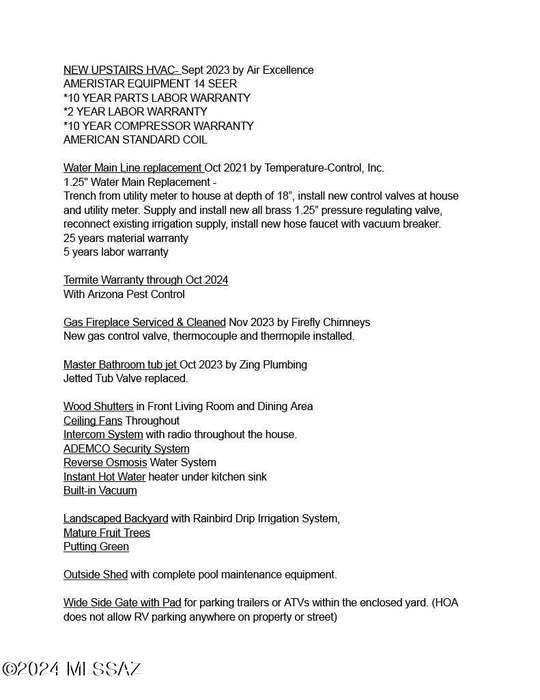The image features a detailed service record in small, easily readable black text, structured into nine sections varying in length. Titled "2024 MESA 7" at the bottom left, it includes an underlined serif heading stating "new upstairs HVAC, September 23, 2023 by Air Excellence." This highlights installations and warranties for Amistar equipment, specifically listing a 14 SEER rating with a 10-year parts and labor warranty, 2-year labor warranty, and 10-year compressor warranty, followed by "American Standard Coil." Further items include a water mainline replacement dated October 2021 by Temperature Control, Inc., describing the technical specifics such as the 1.25-inch water main replacement trench depth, new control valves, and a 25-year material warranty. The record also details other repairs like gas fireplace servicing and bathroom tub jet replacements, suggesting it documents maintenance for an apartment building. The document ends with a footer indicating a 2024 copyright for MESA 7, possibly identifying it as a work order or a service log for a property managed by a company.